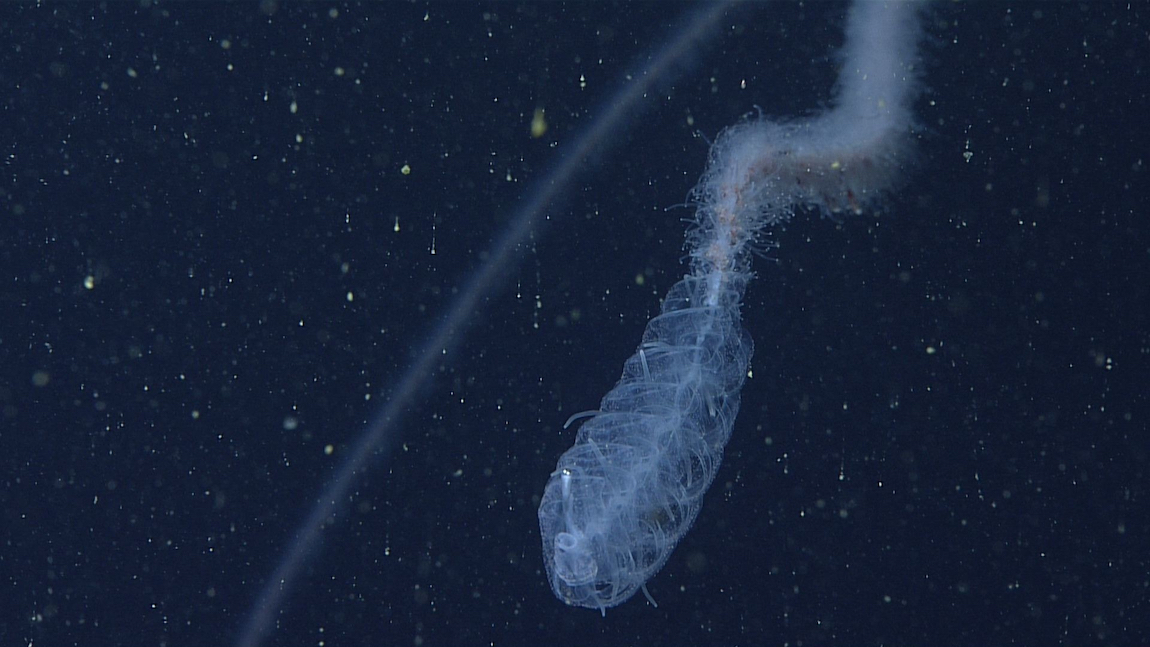The image appears to be an underwater scene or possibly an optical micrograph depicting a dark blue or black field scattered with yellow and white specks that resemble stars or particles. Dominating the scene is a peculiar, transparent creature similar to a jellyfish, situated towards the right. This jellyfish-like organism features fine, strand-like structures resembling a furry tail at the top and other delicate, tentacle-like extensions throughout its body. It extends diagonally across the image, contributing to the intricate and complex fine structures seen within. To the left of this critter, a distinct, diagonal white streak runs through the scene, adding an ethereal element to the already mesmerizing view. The creature’s clear body and the interplay of light and dark hues in the background suggest we are either peering through a microscope in bright field mode or diving deeper into the ocean, where the water grows darker.